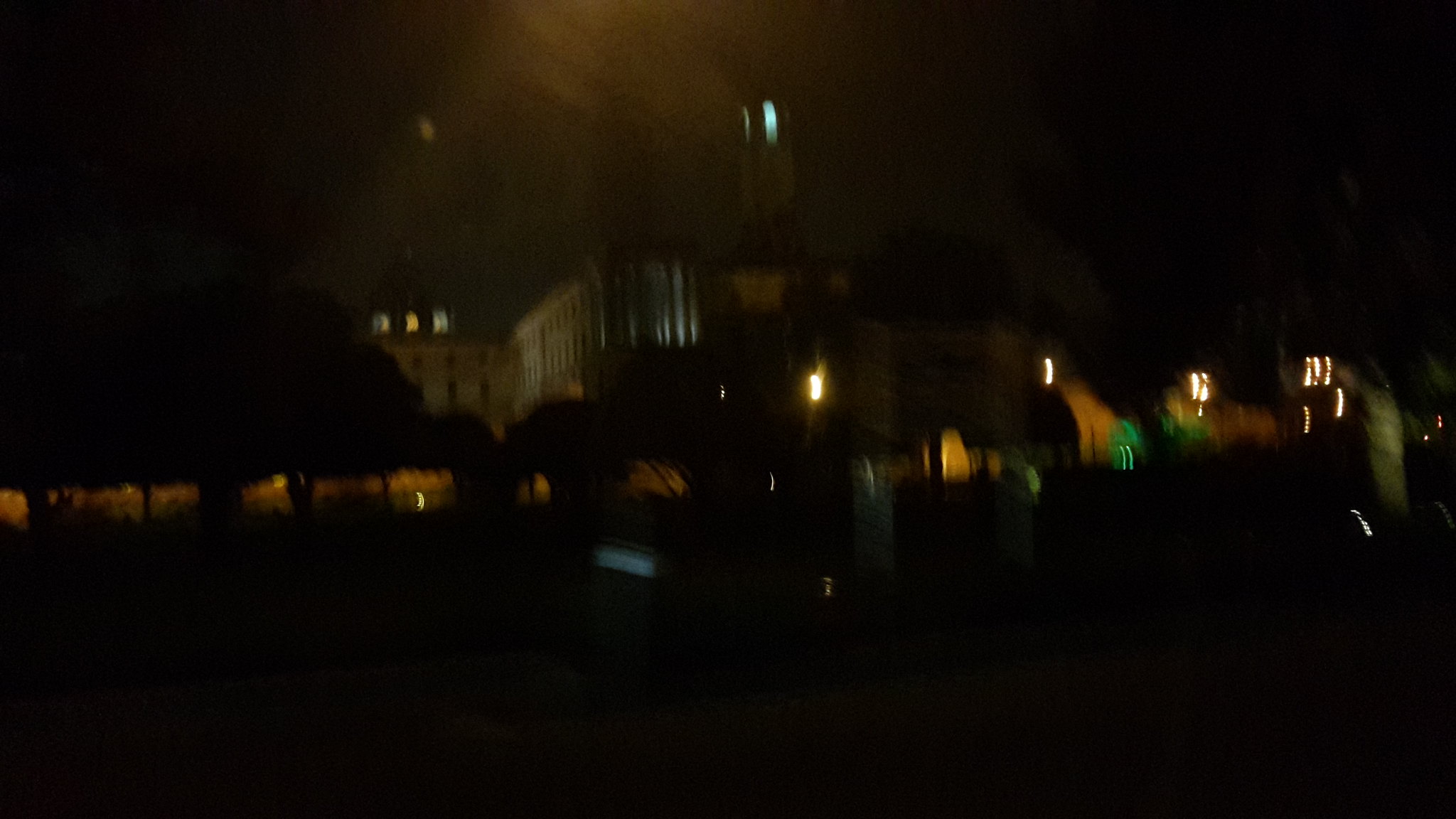This photograph, though extremely blurry and taken from a distance, captures a nighttime scene in a park. In the foreground, a few benches are faintly visible, and an entranceway descending underground can be discerned. The park is surrounded by abundant, tall, and fluffy trees, which obscure much of the view but allow glimpses of large homes or buildings in the background. Due to glare from overhead lights, the scene is bathed in a soft, diffused glow, adding to the overall lack of clarity.

On the right side of the image, the details are almost entirely lost to shadow, with only indistinct shapes providing any context. In the background, partially obscured by the trees, a high-rise apartment building with a brownish-gray facade comes into view. Several of its windows are illuminated, hinting at life within. Dominating the center of the image is a cylindrical tower that extends above the building, though its features remain vague due to the blurriness. Overall, the photograph is an enigmatic and impressionistic portrayal of an urban park at night, with its specific details lost to the limitations of the image quality.